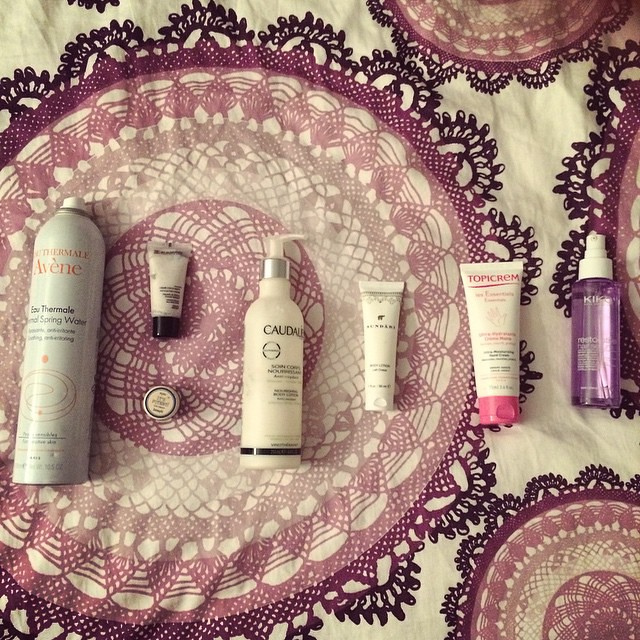The image features an array of healthcare and beauty products laid out on an intricate mat with a mandala-esque design. A pinkish filter envelops the entire scene, adding a warm and cohesive hue. 

From left to right, the items include:
- What appears to be a vein-like object.
- A small circular container.
- A squeeze bottle filled with an unspecified substance.
- A taller bottle partially labeled "Caudel," equipped with a pump dispenser.
- Another squeeze bottle similar to the first one.
- Yet another squeeze bottle.
- Finally, a purple spray bottle.

The mat beneath these items showcases a detailed and ornate pattern, with colors transitioning from bright pinkish-red to dark purple. The careful alignment of the products and the intricate backdrop create a visually engaging and harmonious composition.